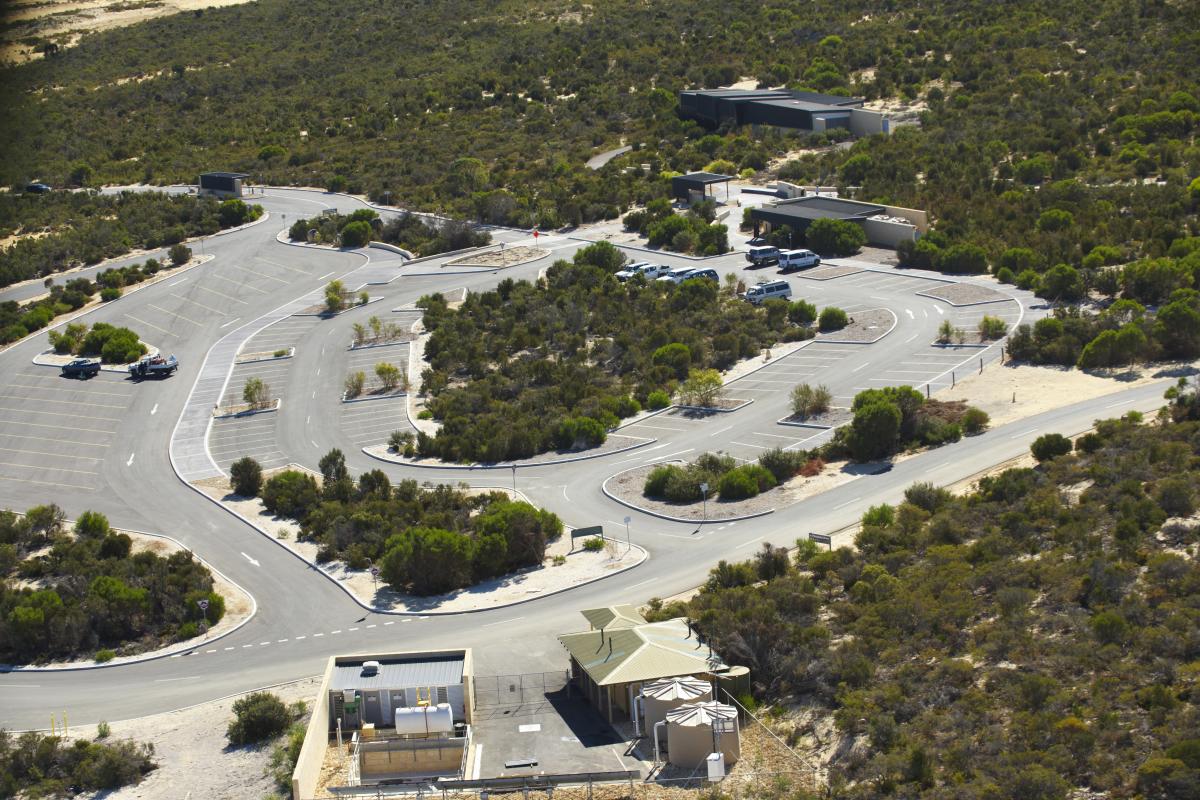This image, captured from a high vantage point, possibly from a plane, showcases an expansive, winding parking lot interspersed with scrub brush and trees. The parking area appears underutilized, with only a few trucks and vans scattered across spaces designed for a much larger capacity. Several low-rise, industrial-esque buildings, including what seems to be a black structure, are visible among the greenery, hinting at a research facility or possibly a water treatment plant. The scene is relatively devoid of pedestrians, suggesting it is primarily a worker area, located seemingly in a remote or isolated region, potentially resembling the California landscape due to the prevalent dry, brown ground speckled with green bushes. At the upper left corner, an entry point resembling a toll booth suggests a restricted access area. The middle front section features a small propane or water treatment shed, further emphasizing the industrial nature of the site. The overall ambiance is one of sparse human activity amidst a predominantly wooded, undeveloped expanse.